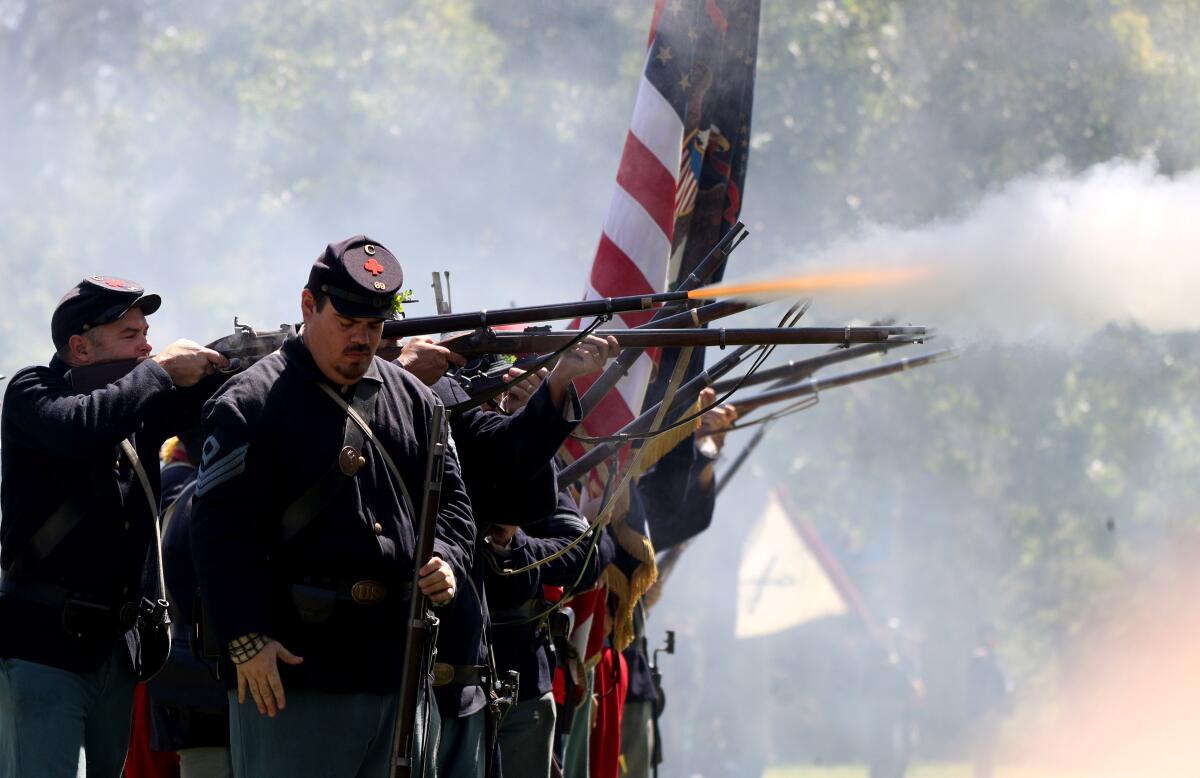The image captures a vivid Civil War reenactment scene featuring Union troops standing shoulder-to-shoulder in a single-file line. The soldiers are dressed in traditional blue uniforms with matching blue hats that feature a red cross symbol on top. There are at least ten muskets or rifles in various stages of use, adding to the authenticity of the scene. A dramatic muzzle flash is visible from one of the muskets, and the area is enveloped in a thick cloud of smoke from the gunfire. A large American flag and another flag, possibly with crossed swords, flutter in the background, partially obscured by the smoke. One man in the foreground stands out; his rifle is propped beside him as he appears to be checking his pockets, possibly searching for something. His downcast expression adds a somber tone to the scene. The backdrop of green-leaved trees is faintly visible through the haze, contributing to the historical ambiance.